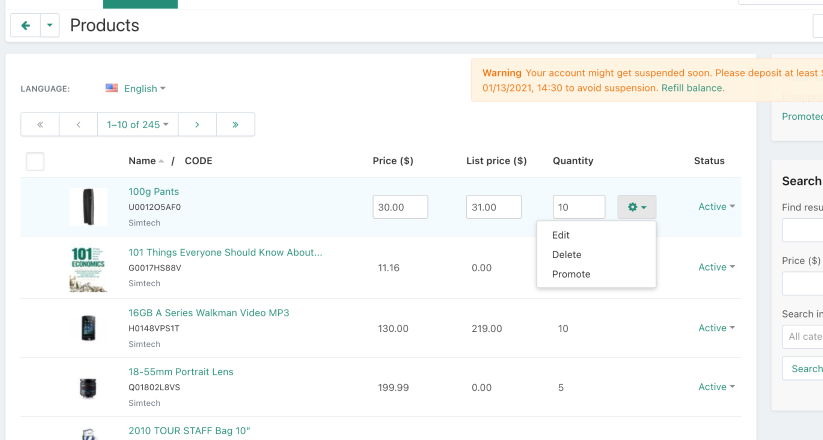The image is a detailed screenshot of a shopping website interface with a white background and a gray border. 

In the top left corner, there's a green leftward facing arrow icon, followed by a downward facing green arrow. To the right, the word "Products" is displayed in dark gray. Slightly above "Products," there is a horizontal green rectangle.

Further down, on the left side, it says "Language" in light gray, accompanied by an American flag icon. To the right of the flag, "English" is written in light blue with a downward facing arrow.

On the right side, there's a peach-colored horizontal rectangle. Inside it, "Warning" is written in bold orange letters. Below that, in regular letters, it reads, "Your account might get suspended soon, please deposit at least," but the text is cut off. Underneath, it says, "1-13-2021-1430 to avoid suspension," all in orange. To the right of this message, "Refill Balance" is written in blue.

Moving further down, a short list is presented. It includes a dark gray leftward facing arrow and a light gray leftward facing arrow. In the middle, it says "1-10-245" in blue with a downward facing arrow. To the right, there is a light blue rightward facing arrow, and furthest to the right, there is a double rightward facing arrow.

Beneath this, a highlighted column displays product details. There is a small image resembling a black vertical rectangle. To its right, "100G Pants" is written in light blue. Below that, "U001205AFO" is in black, followed by "SimTech" in gray. Further to the right, in the price category, it says "$30," and in the list price category, it says "$31." In the quantity category, it lists "10." To the right, there is a settings button and a downward facing arrow button. The dropdown menu includes options to "Edit," "Delete," and "Promote," all in dark gray. Furthest to the right, in the status area, it says "Active" in blue with a downward facing arrow button.

The next row features a thumbnail image labeled "101 Electronics," depicting various electronic devices in the background. To its right, "101 Things Everyone Should Know About" is written in blue. Below it, "G0017HSB8V" is in black, followed by "SimTech" in gray. Further to the right, in the price category, it lists "$11.16," and in the list price category, it states "$0." The quantity category is obscured by an overlapping box from above with "Edit," "Delete," and "Promote" options. Furthest to the right, the status reads "Active" in blue with a downward facing arrow.